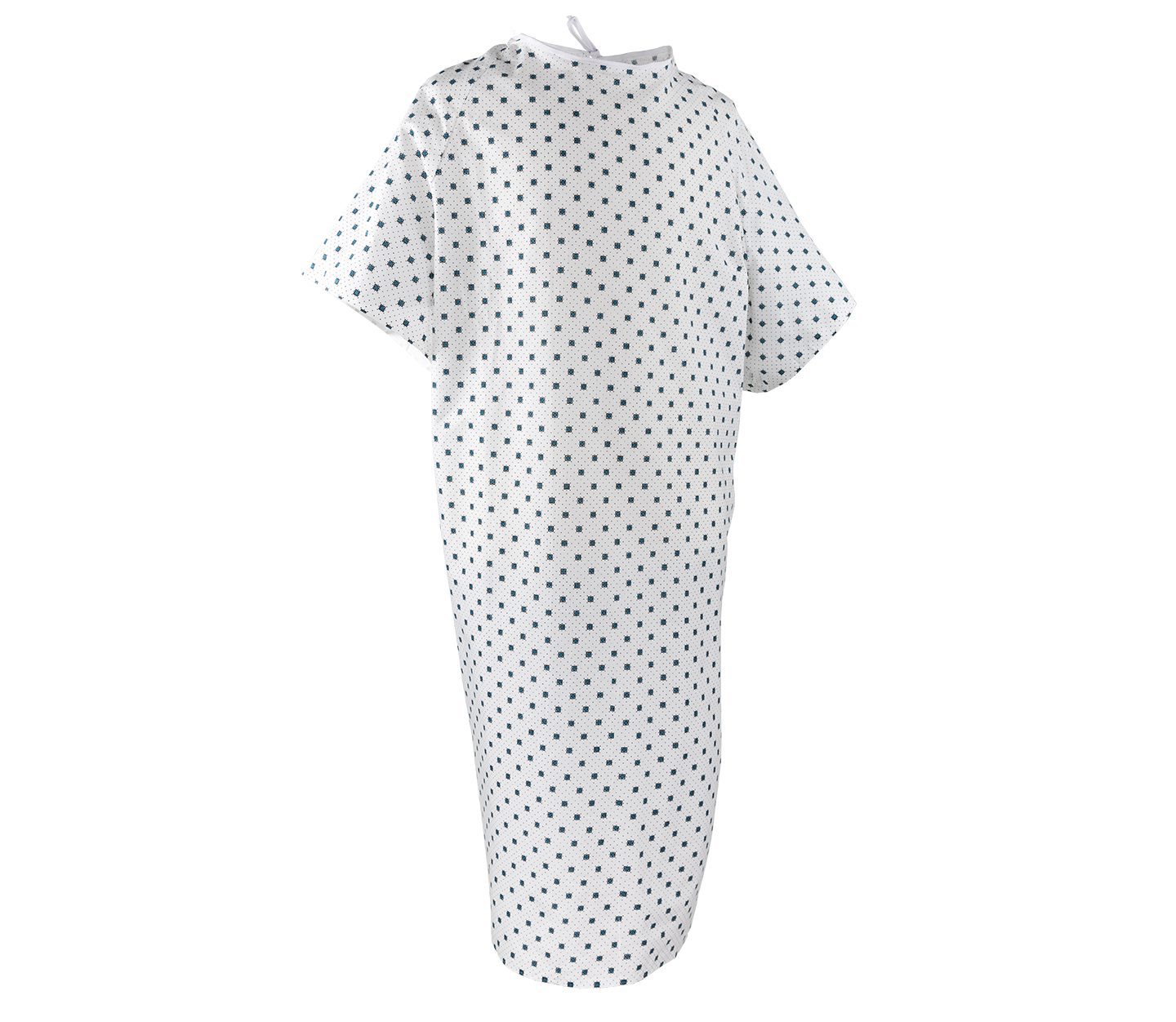This image features a typical adult hospital gown displayed on a purely white background, with no mannequin or hanger visible. The gown is predominantly white, adorned with a pattern of small, dark blue squares arranged in a consistent, diamond-like pattern throughout the fabric. It is a wraparound style and appears to tie at the neck in the back. The gown has short sleeves, a fairly wide neck opening, and wide arm sleeves. It is designed to reach approximately mid-shin on an adult. Overall, the gown portrays the standard, simple design commonly seen in hospital settings, and is likely made of cotton.